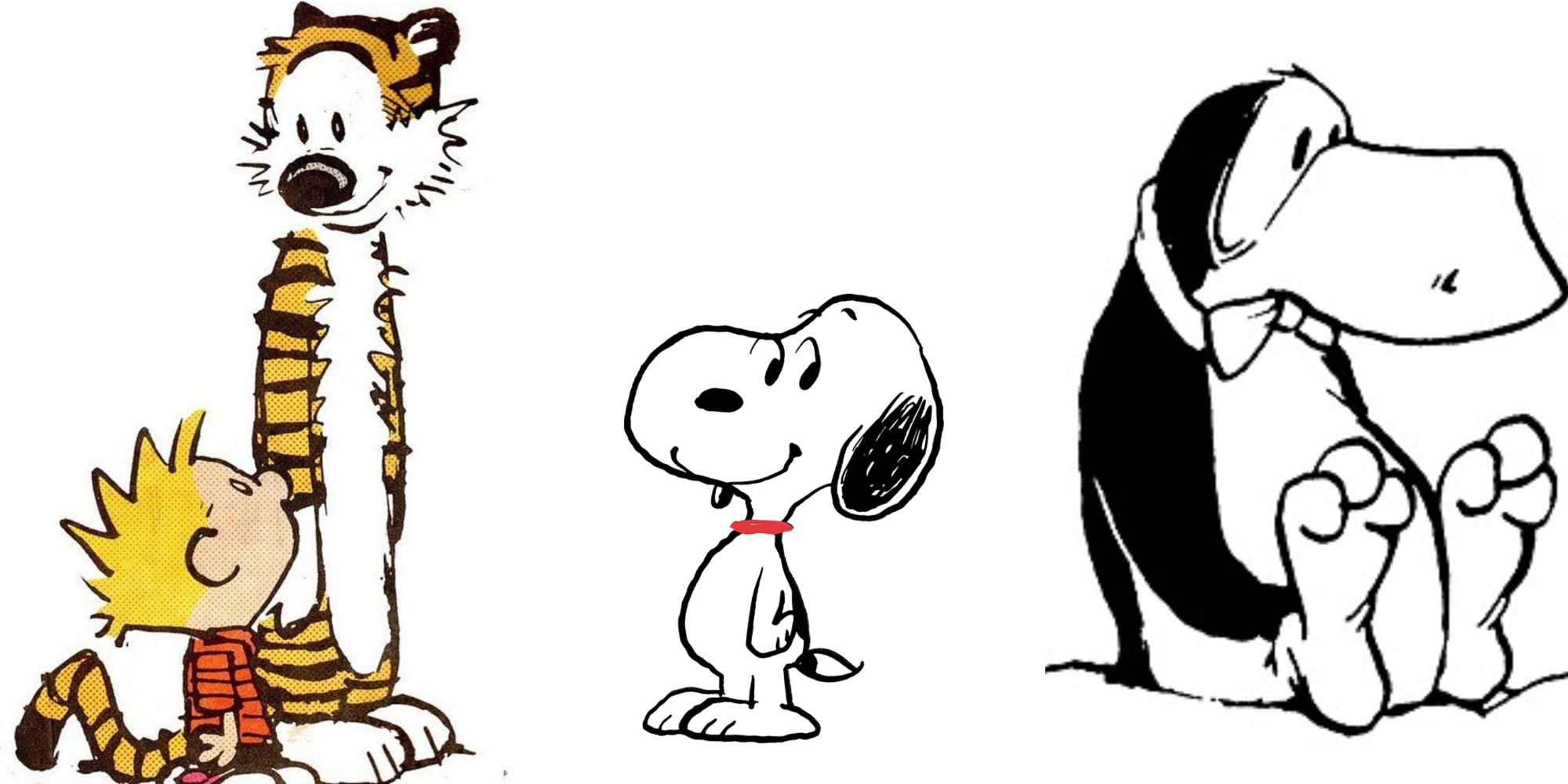The image depicts three distinct cartoon characters from classic comic strips. On the left, Calvin and Hobbes are vividly illustrated in color. Calvin, a little boy with spiky blonde hair, is wearing a red striped shirt and white and red shoes, and is shown looking up at his stuffed tiger, Hobbes, who appears as a real tiger with orange and black stripes, taller than Calvin. In the center is Snoopy from the Peanuts comic strip, characterized as a black and white beagle, smiling and wearing a red collar. On the right is an intriguing black and white character that resembles a penguin, with a single large eye, sitting and gazing into the distance. This final character's name is uncertain, referred to as possibly Filbert or Bilbert. These three images together evoke the charm and nostalgia of beloved Sunday comic strips.